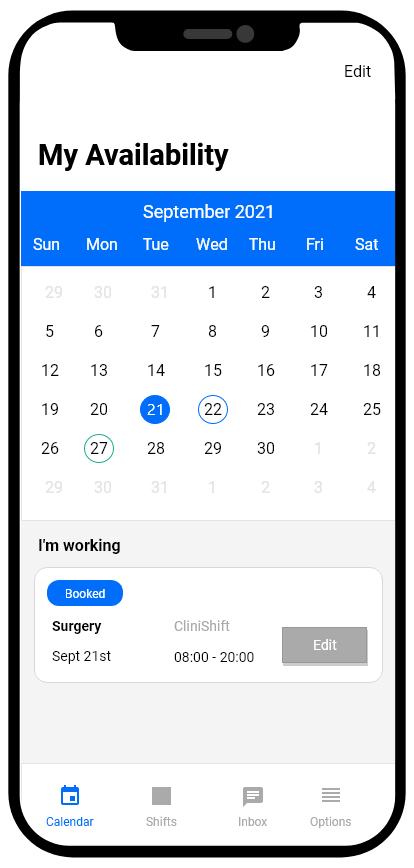Screenshot of a cell phone display showing a user’s availability calendar for September 2021. In the upper right corner, there is an "Edit" option. Below and to the left in black text, it says "My Availability." Beneath this, a blue bar extends horizontally with "September 2021" written in white. The days of the week—Sunday through Saturday—are listed in a row.

The subsequent section shows a calendar grid. The displayed days span from August 29 to October 2, detailing each day's number. Notably, the 21st and 22nd are highlighted with blue circles, while the 27th is marked with a green circle.

Under the calendar, the text "I'm working" is displayed in black. Beneath it is a blue "Booked" button. Following this, "Surgery and Clinic Shift" is noted, specifying the work date as "September 21st, 8 a.m. to 8 p.m." 

The gray "Edit" button with white lettering appears next to this information. At the bottom of the screen, a navigation bar lists "Calendar," "Shifts," "Inbox," and "Options" (represented by a menu icon with three or four lines).